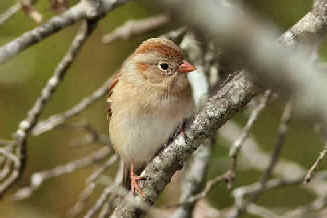This is a close-up outdoor image featuring a tiny, puffy bird perched on a grayish-brown branch that stretches diagonally from the upper right corner to the lower left. The background is a blurred mix of green and hints of orange, suggesting a natural setting filled with foliage and trees. The bird, positioned centrally, has soft red feet and a delicate beak of the same color. Its head, turned slightly to the right, showcases a distinctive gold-gray hue with a darker brown streak across the top. The bird's body transitions from light brown to an almost white underbelly. Its black eyes are encircled by a fine white ring, giving it a sweet and endearing appearance.